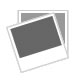The image depicts a vintage sign shaped like an old dress shoe, designed to advertise a shoe repair service. The sign is predominantly brown with a mixture of dark and light brown shades. The sole of the shoe is dark brown, while the main body features both dark brown and light brown sections. The heel and toe areas are dark grayish blue, bordered with teal trim. The shoelaces are green with brass rings around the eyelets, and the text "SHOE REPAIRING" is prominently displayed in beige, capital letters on the shoe’s upper part. On the right side of the shoe, which is the back, there are two metal rods with drilled holes—for mounting purposes—extending from the top and bottom. Additionally, a single metal rod protrudes from the front of the shoe, likely intended for hanging the sign on a wall. The background of the image is plain white, making the detailed and colorful sign stand out.